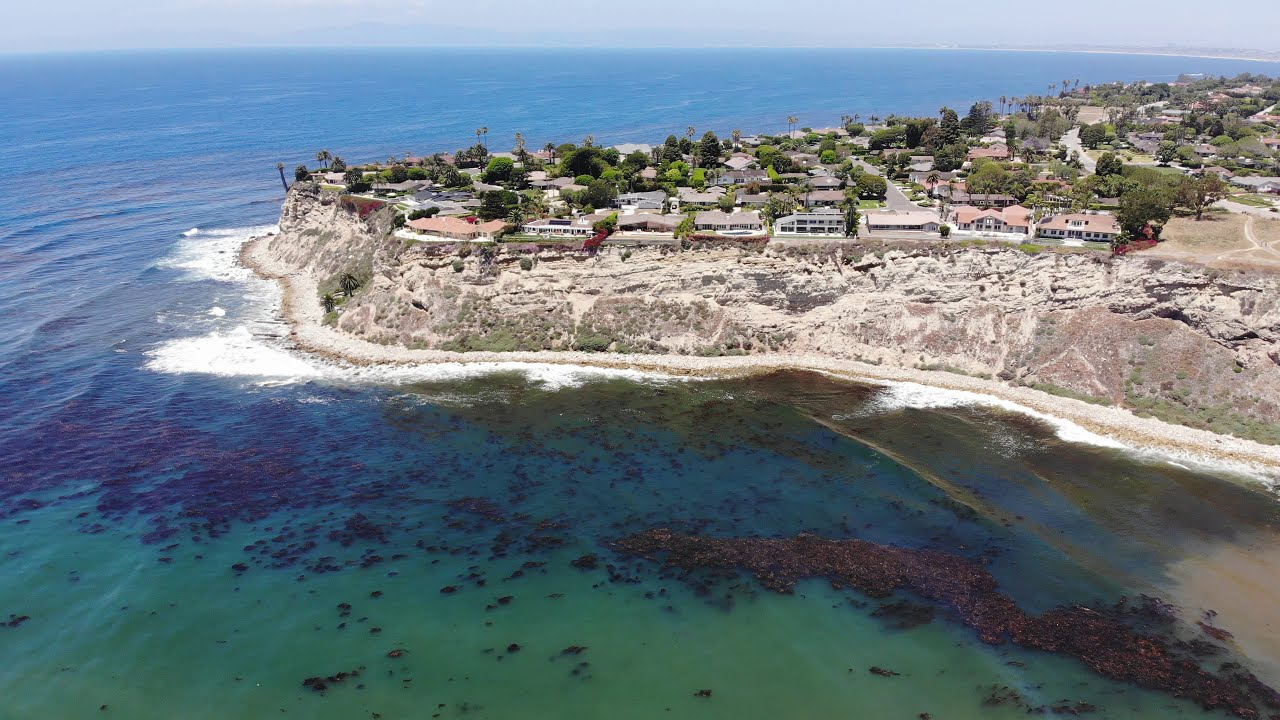This is an aerial daytime photograph capturing a rugged island protruding into the ocean. The island is characterized by a cliff face, making direct access to its rocky beach below quite challenging. Dominating the island are various houses, predominantly one-story with distinctive red roofs, though a few two-story structures stand out. Among the buildings, green trees are interspersed, adding to the island's charm. The ocean surrounding the island exhibits a gradient, with darker waters near the cliff and greener hues towards the bottom of the image. The waves crash against the left side of the land, creating white foam amidst patches of black algae. In the distant background, faintly visible outlines of mountains add depth to the scenery. The entire scene is framed within a horizontal rectangular layout, with the horizon line running straight across the upper part of the image.